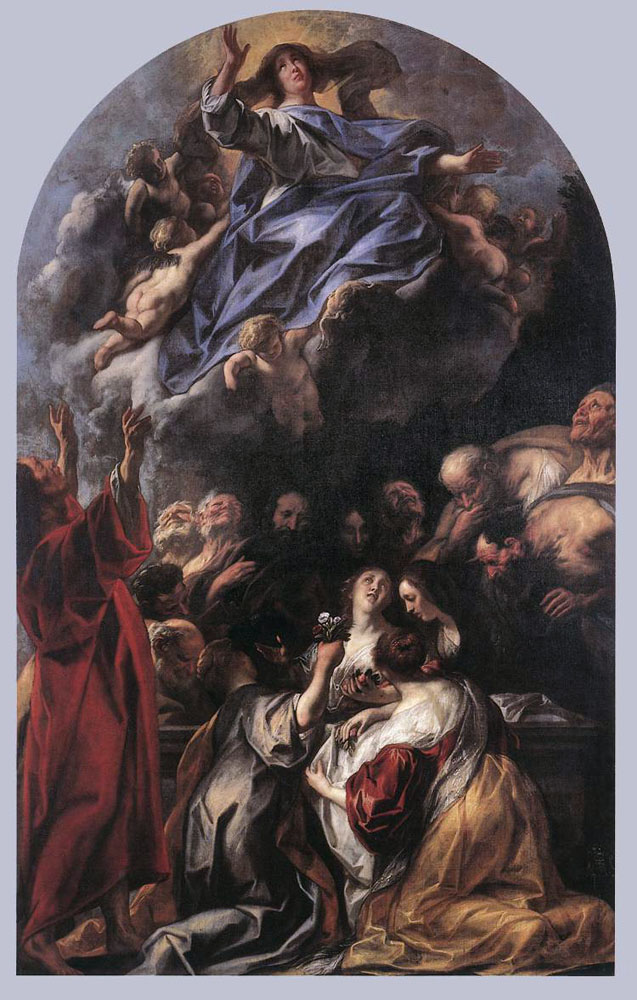The painting portrays a heavenly ascension scene, featuring a central holy figure surrounded by a multitude of baby cherub angels. The central figure at the top, who appears to be a woman, is wearing a flowing blue gown and holds her hands raised upwards towards the heavens. This figure is illuminated, emphasizing her divine ascent amidst billowing dark gray clouds. Below her, multiple adult figures, approximately ten in number, are depicted in various states of prayer, concern, and grief. Central among them is another woman in a red gown and a white robe, who appears to be looking up at the ascending figure, possibly being attended to or consoled by those around her. The setting is framed with a painted arch and the background is a dusty light blue, giving the piece a serene yet somber ambiance. The detailed composition conveys a sense of worship, divine intervention, and human concern, reminiscent of classical masterpieces by renowned artists.